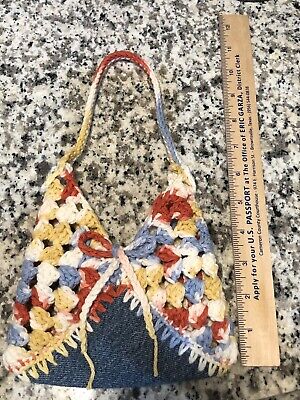The image features a handcrafted purse resting on a grey, black, and white marbled countertop. The purse is distinctive with a knitted upper portion and a triangular bottom made from dark blue denim. The knitwork exhibits a variety of colors, including blue, white, red, and orange, intricately woven and braided together. A bowtie, fashioned from a crocheted chain, decorates the center front of the purse. The bag sides exhibit a textured granny square stitch design, while the handle appears to be single crochet. Next to the purse on the right side is a wooden ruler, which features the text "Apply for a U.S. passport at the office of Eric Garza" and measures the purse's total length at 11 inches.